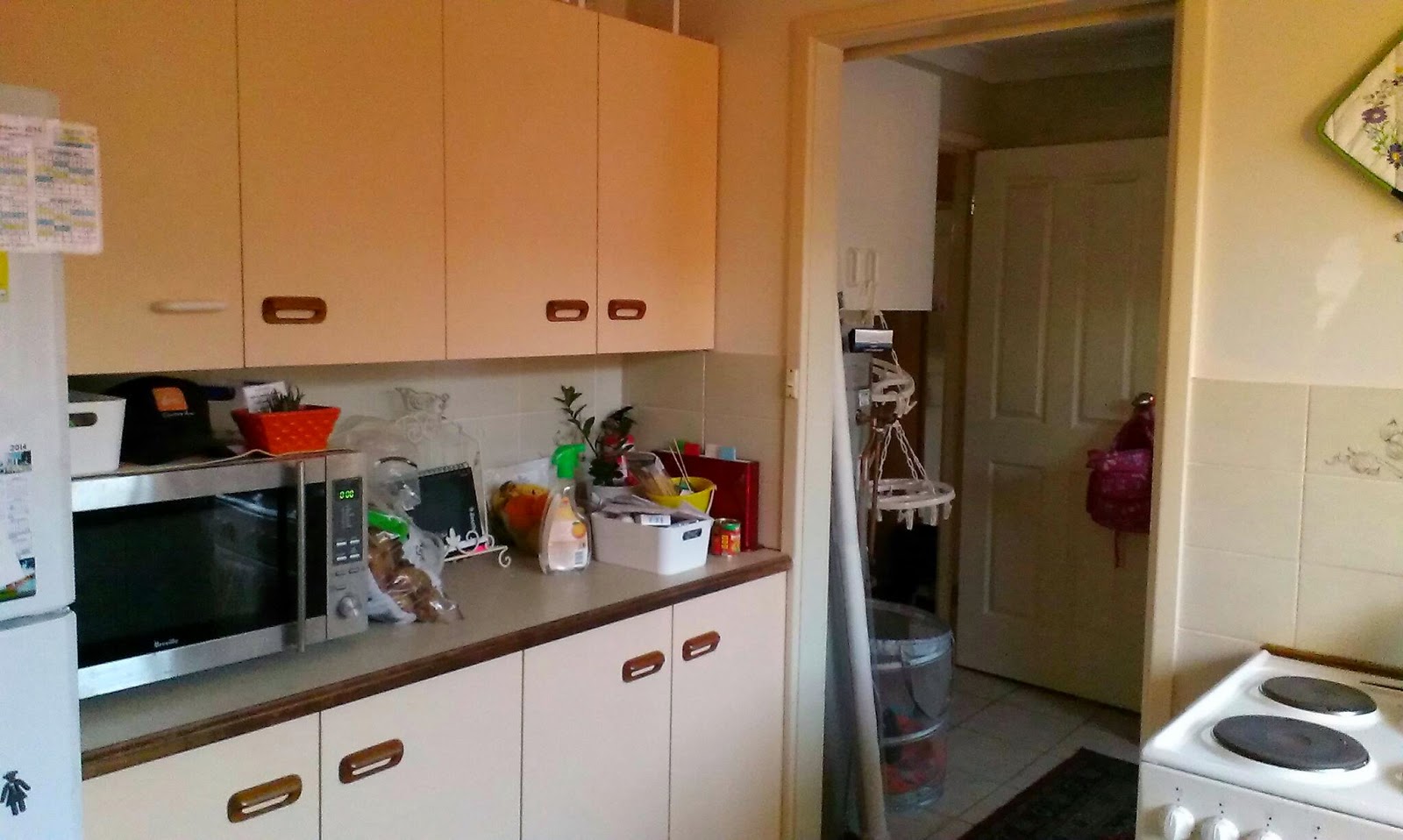The image depicts a cluttered kitchen with limited counter space. To the right of a white refrigerator adorned with magnets, a microwave is precariously placed, leaving only about four to five inches of counter space in front of it. The countertops appear to have an orangey hue, possibly due to sunlight, but likely match the off-white cabinets that feature brown plastic handles. The counter is crowded with various items, contributing to the overall sense of disarray.

Beyond the kitchen, an open door reveals what resembles a laundry room, containing a couple of counters with different handles and a floor mat. Adjacent to this door on the right is an electric stove, which has plain, lid-covered burners and controls located on the front. The presence of an oven is assumed but not visible in the image. The kitchen as a whole appears dated and in urgent need of renovation.